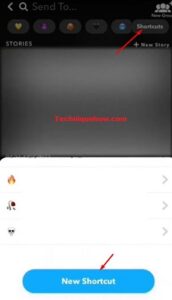The user interface of a social media application is displayed, featuring a variety of icons, options, and labels. At the top, a back arrow is visible next to a search bar accompanied by an option labeled "Send to," indicating the functionality to send items to specific usernames. Adjacent to these are a "New Group" option with multiple people icons, suggesting the ability to send messages to multiple recipients.

Below these elements, there is a sequence of colorful icons: a yellow heart, a purple circle, a brown circle, a black heart, and a blue circle, all alongside an option for "Shortcuts" indicated in white text, with a prominent red arrow pointing toward it. Beneath this section, "New Story" is presented in bold white letters accompanied by a white plus sign.

On the left, the word "STORIES" is displayed in capital white letters. Below this label lies a square gray space with indistinct red writing at its center, rendered unreadable due to blurriness. Further below, a fire icon graces the leftmost side, followed by white space and an arrow. Adjacent to it is an icon resembling a wilting rose, drooping to one side, accompanied by white space and an arrow. Another icon follows, depicting a white skull with dark black eyes, set beside white space and an arrow.

At the bottom of the interface, "New Shortcut" is written in white letters, nested within a filled blue border. A small red arrow points directly to the "New Shortcut" text, indicating its position.

This detailed visual arrangement encapsulates the various navigational and interactive elements available within the social media application's interface.